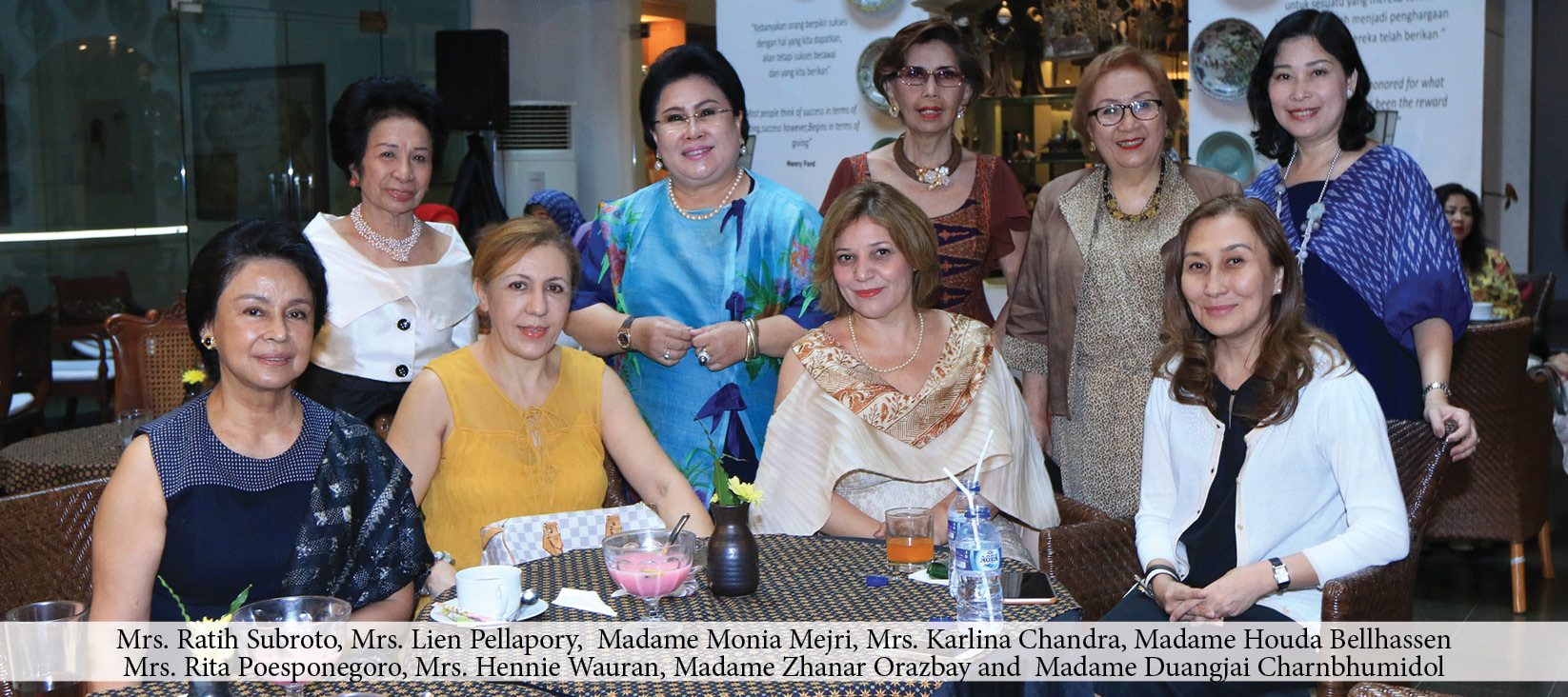This is a wide, horizontal, rectangular image capturing a formal gathering of nine middle-aged women in a restaurant. The image shows four women seated at a round table adorned with a patterned gold and black table cover, while five women stand behind them. They are all dressed formally in a variety of colored tops—white, light blue, brown, white-brown, light and medium blue, dark blue, medium yellow, tan, and white—and are smiling at the camera. In front of the seated women, there is a table with a bowl containing something pink, a couple of bottles of water with straws, and a glass of orange juice. In the background, two large screens, which could be menu boards or projection screens, add to the restaurant ambiance. At the very bottom of the image, in a small light gray rectangular section, their names are listed in black text: Mrs. Rati Subrato, Mrs. Lene Pelopori, Madam Monia Mejri, Mrs. Karleena Chandra, Madam Huda Belhassen, Mrs. Rita Paz-Pinagoro, Mrs. Hennie Warren, Madam Zanar Al-Razbeh, and Madam Duongjai Sharnabhumidul.